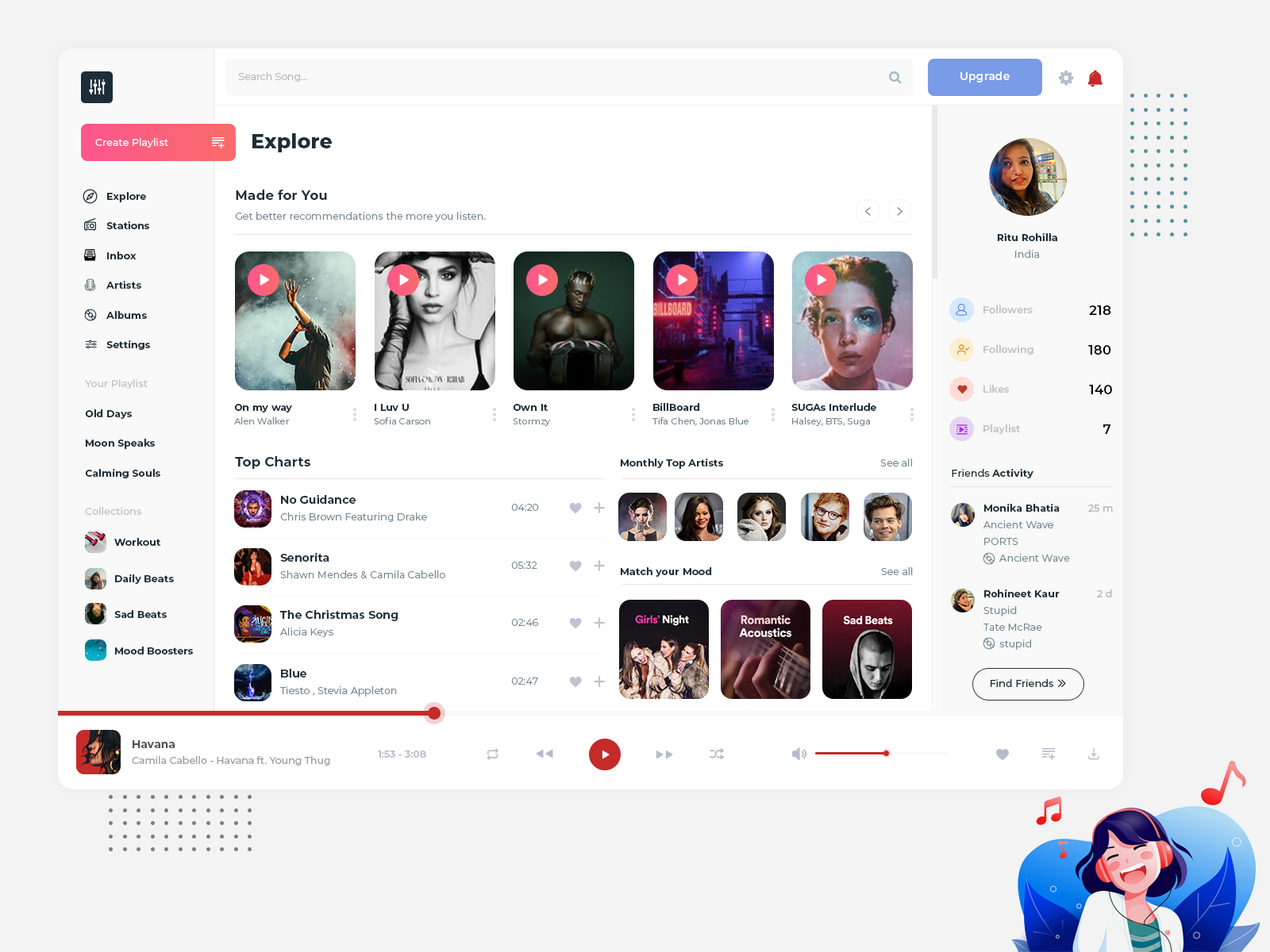**Detailed Caption:**

The image displays a user interface with a white background encompassing the entire screen. In the top left corner, there is a square button. Directly below this, there is a pink box that reads "Create Playlist." Following this, the text "Explore Stations," "Inbox," "Artists," "Albums," and "Settings" are listed sequentially.

Further down, the interface showcases a section titled "Playlist" that features several album titles: "Old Days," "Moon Speaks," "Calming Souls," and an indistinguishable title. Below this, additional playlists are named: "Workout," "Daily Bears," "Sad Bears," and "Mood Boosters."

In the center of the page, the heading "Explore" is displayed, followed by the subheading "Made for You." Beneath this, there are album covers organized in rows, each accompanied by a play icon. The albums' titles, listed from left to right, are as follows: "On Anyway," "I Love You," "Own Be," "Billboard," and "Why Gilba? Interlude."

Below this section, there is a "Top Charts" area filled with thumbnail icons of various albums, along with their respective names and artists. To the right of the "Top Charts" section, the screen showcases another area labeled "Monthly Top Artists," followed by a section titled "Match Your Mood."

On the far right side of the interface, there is a blue "Upgrade" button with white text. Underneath this button, an icon of a person appears along with the individual's name and their statistics for the website.